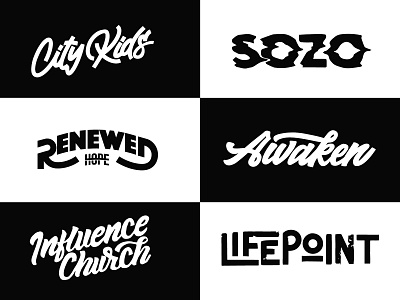The image showcases six rectangular logos arranged in three rows of two. The top row features a black-background rectangle on the left, with the white script text "City Kids" angled upward. To its right, on a white background, is the logo "SOZO" in jagged black capital letters. The middle row starts with a logo on a white background, "RENEWED HOPE" in black capitalized letters, with "RENEWED" on the top line and "HOPE" in smaller letters below, and stylized extensions from the R and D underlining parts of the word. Beside it is a black-background logo with the word "AWAKEN" in white cursive. The bottom row has on the left, a black rectangle with "INFLUENCE CHURCH" in angled white cursive, and on the right, a white-background logo with "LIFE POINT" in black letters, featuring an extended L that underlines “IFE” and an O in "POINT" that's smaller with an underline beneath it.